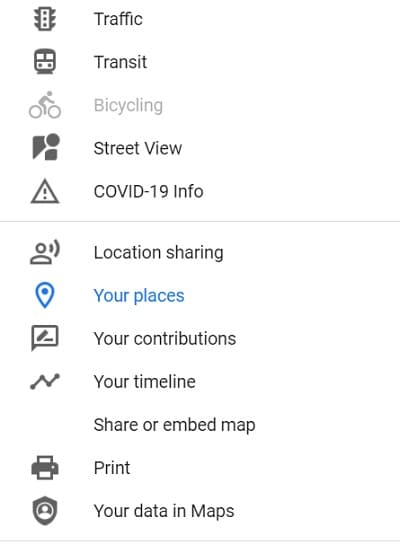The image depicts a webpage or a smartphone website interface with a white background and a list of options written in dark gray text. Each option is accompanied by a small symbol on its left. The detailed list from top to bottom includes:

1. A traffic light icon followed by the word "Traffic".
2. A bus icon next to the word "Transit".
3. An icon of a bicyclist paired with the word "Bicycling".
4. The Google Maps Street View symbol alongside the words "Street View".
5. A yield warning sign (a triangle with an exclamation point) beside the words "COVID-19 info".
6. An icon depicting a person with a hearing aid denoted as "Location sharing".
7. The words "Your places" in blue.
8. A message box icon with a pen next to the words "Your contributions".
9. An icon resembling a bar graph labeled "Your timeline".
10. The text "Share or embed map".
11. A printer icon beside the word "Print".
12. A badge icon with a person symbol and the words "Your data in Maps". 

This interface likely belongs to a navigation or maps application, providing various features and information for users to interact with.